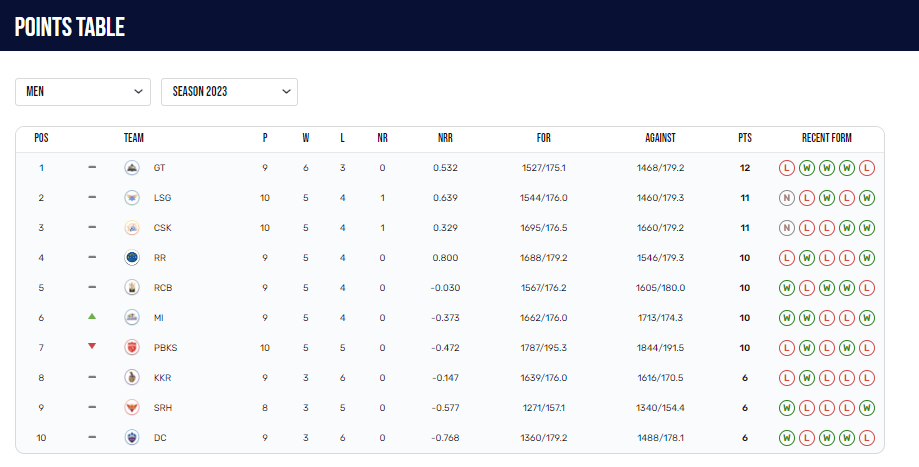The image displays a comprehensive points table for the 2023 season. The table is prominently labeled "Points Table" in white text on a dark blue background. The main section of the table is set against a white backdrop with black text and includes various filters for customization. 

At the top, there are options to toggle between different categories, indicated by the label "Men" and an adjacent arrow icon, suggesting additional filters are available. The season is clearly specified as "2023," accompanied by a drop-down arrow for selecting different seasons.

The table features detailed statistics for 10 different teams, organized into several columns. These columns include the team's position, name, matches played, wins, losses, no-results, and abbreviations like NRR (Net Run Rate). Additional columns such as 'For,' 'Against,' and 'Points' provide further insights.

The 'Recent Form' column uses color-coded circles to represent each team's performance: green for wins, red for losses, and gray for no-results. The top-ranked team leads with 12 points, while the team in the 10th position has 6 points.